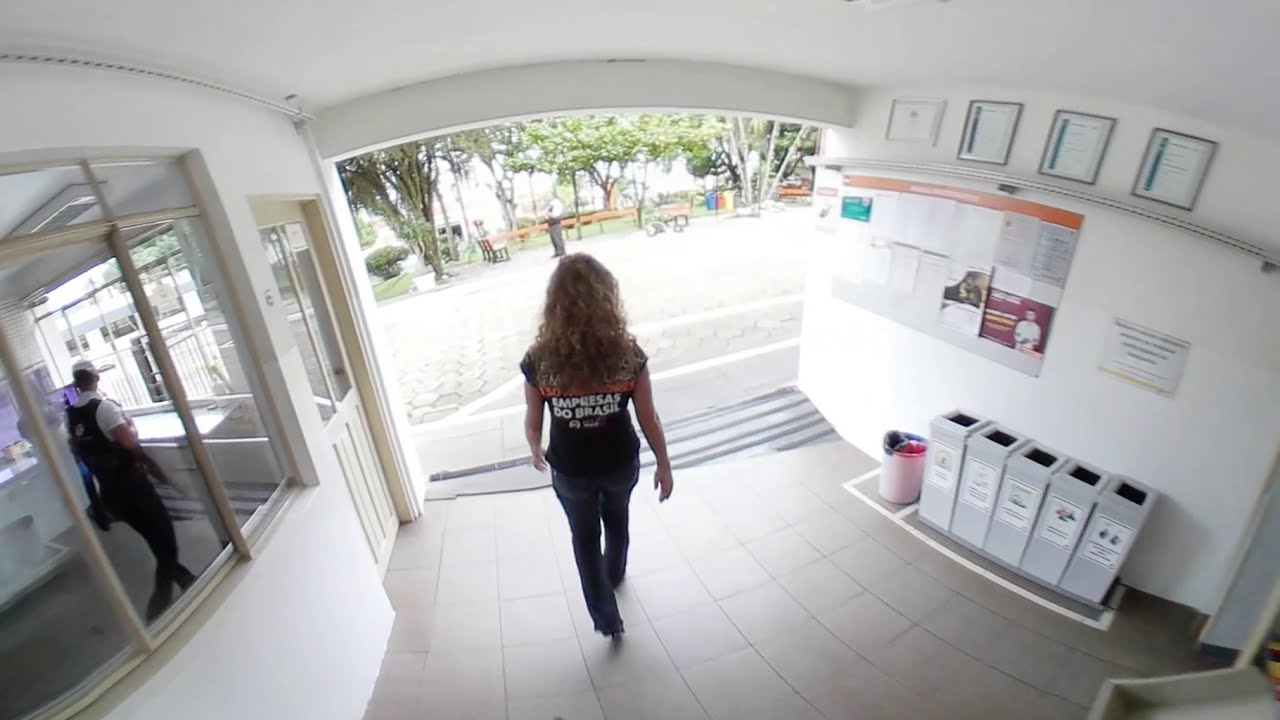This photographic image captures an indoor setting, focusing on a blonde woman who is walking down a hallway towards an outdoor patio or cobblestone walkway. She is wearing dark pants and a black t-shirt with white text that reads "EMPRESAS DO BRASIL." To the right of the image, along the wall, there are various bins including recycling and trash bins, along with a series of plaques, frames, and an unreadable poster with multiple colors, believed to be in orange, green, and red. Additionally, five long rectangular boxes with holes are positioned below the frames, with a red bucket next to them. On the left side, there is a white door with glass panes, leading into a store where a man wearing a white baseball cap, white t-shirt, black pants, and carrying a black vest is visible. The hallway seems to lead outdoors where green trees and park benches can be seen, along with a person standing up. There are also visible large blue, red, and yellow recycling buckets outside. The building has an open entryway without a front door, enhancing the corridor’s transition from indoors to the outdoor patio area.